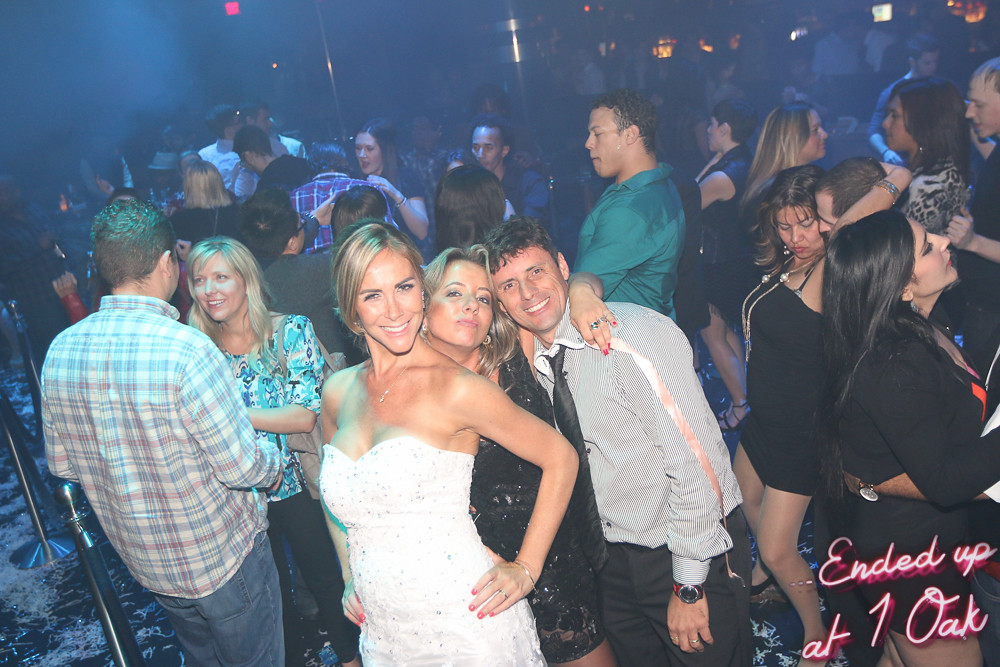The image depicts a lively scene at a nightclub, potentially a wedding afterparty, as suggested by the celebratory atmosphere and the attire of the individuals. Front and center, three people are prominently posing for the camera. On the left is a smiling blonde woman in a white dress, possibly a wedding or party gown. Next to her, a woman in a sparkling black dress is making duck lips, while a man on her right wears a gray, striped button-down shirt, black tie, and slacks, with a wristwatch on his left hand. The background is filled with people dancing and interacting, including a man in a teal shirt and a woman in a black mini dress dancing close to a partner. The room has a somewhat smoky ambiance, and various colors are visible amid the crowd, including black, white, gray, silver, hot pink, red, teal, blue, and brown. In the lower right-hand corner, neon pink cursive text reads "Ended up at One Oak." The overall composition and details suggest a vibrant nighttime celebration at a popular club.